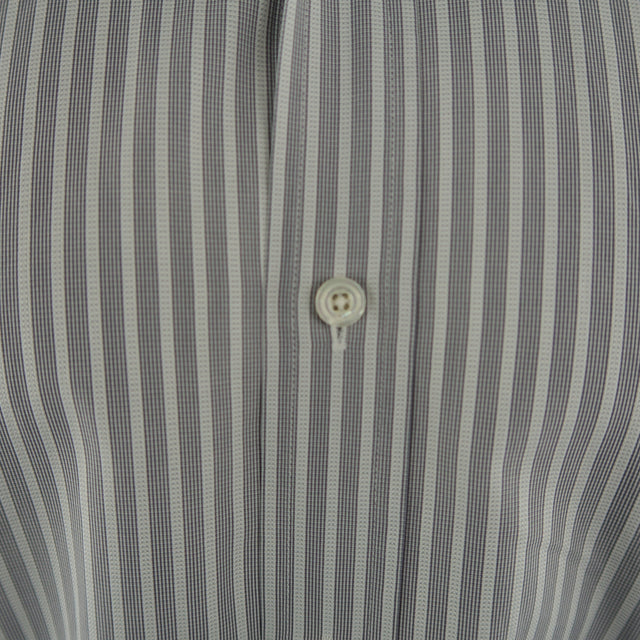The image is a detailed close-up of a section of a men's dress shirt. The shirt features horizontally woven texture and distinct stripe patterns of varying shades of gray. The darker gray stripes are about twice as thick as the lighter gray ones, adding depth to the fabric. The shirt appears to be finely pressed, possibly with starch, accentuating the crisp detail. In the center of this section, there's a single, shiny white button with four small holes, secured with light gray stitching that blends harmoniously with the fabric. The button and buttonhole, reinforced to prevent fraying, add to the meticulous craftsmanship of the shirt. The textured fabric and the intricate weave pattern, along with the mother-of-pearl shimmer of the button, highlight the quality and attention to detail in the design.